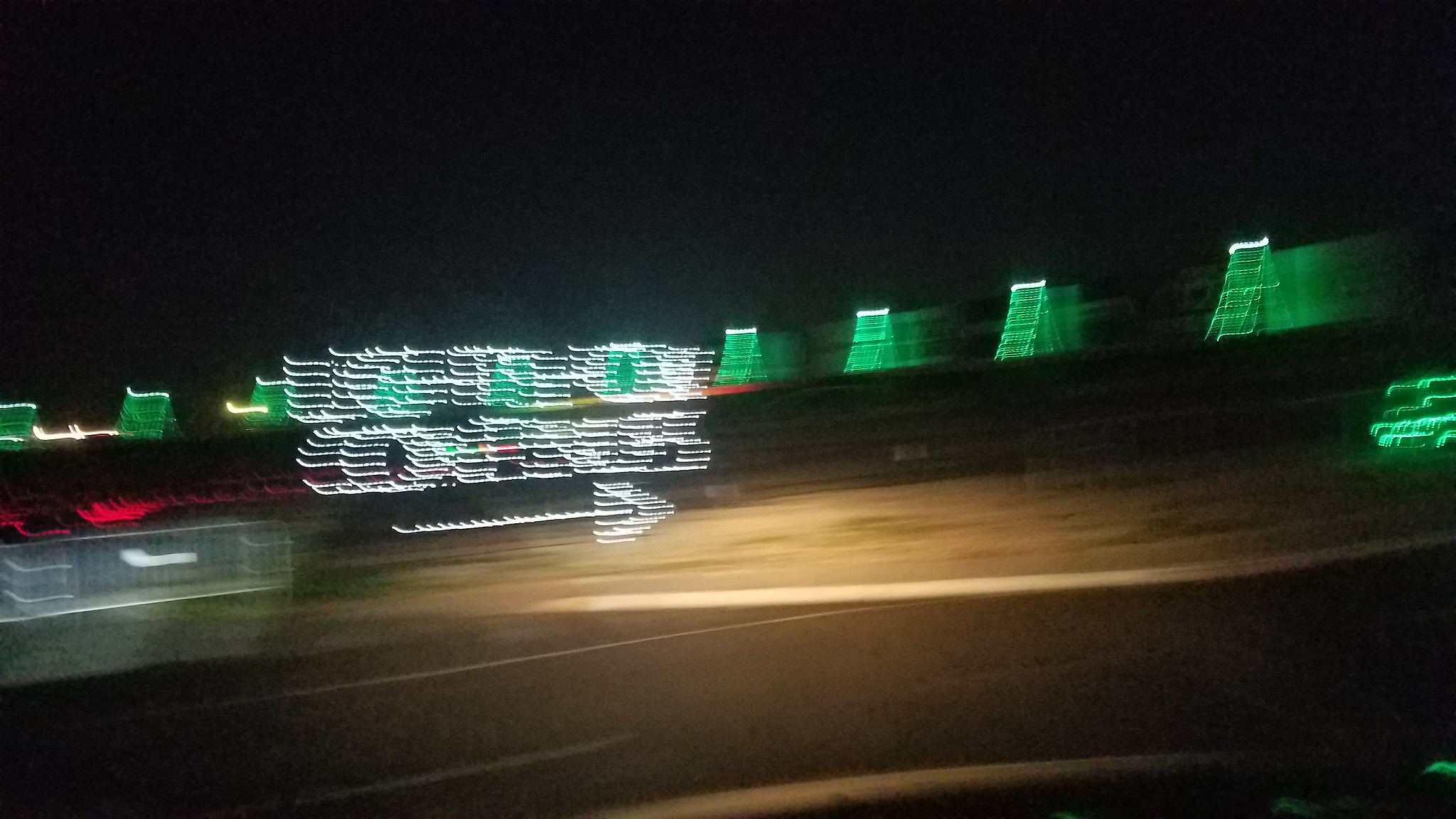A nighttime photograph taken from a moving vehicle captures a scene filled with blurred and out-of-focus elements, indicative of high-speed motion. Dominating the image, white signage with illegible text due to motion blur appears in the center, accompanied by a right-pointing arrow below it. The background features a row of lit green, triangular shapes lining the top edge from left to right, possibly suggesting the illuminated border of a building or stadium. Below the signage, a field with a mix of dirt and sparse grass is visible. In the foreground, a tarred road with faintly visible lane markings leads towards a rectangular structure bathed in white lights on the left side, giving the appearance of a cage. The entire scene is heavily distorted, conveying a sense of movement and obscuring clear details.